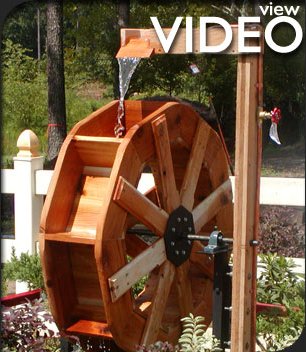The photograph showcases a detailed scene of a wooden water mill in action. The mill consists of a light brown, slightly orange-tinted wooden wheel with small rectangular openings spaced throughout. Water drips from an upper brace into the wheel, causing it to turn. Additionally, a wooden post extends horizontally and is designed with an element that allows water to drain into the large wheel. Surrounding the mill is a garden area dotted with various plants and greenery. In the background, a low white picket fence with horizontal slats delineates the boundary. Beyond the fence, tree trunks and dense brush add depth to the scene. Prominent white lettering on the image reads "view video," with "view" being smaller and "video" larger, enhancing the overall setting and picturesque quality of the photograph.